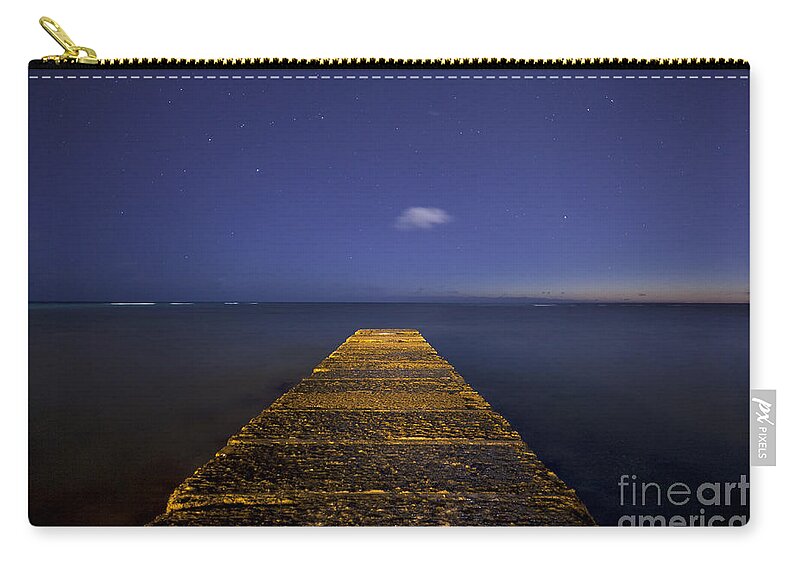This image showcases a striking fine art painting displayed on a rectangular, flat zipper pouch. The pouch features a shiny brass zipper running across the top, and the case has three sides. The smooth surface of the pouch is set against a white backdrop. The focal point of the painting is an old, weathered wooden pier with no railings, stretching out into dark, murky water. The planks of the pier appear rough and aged, transitioning from a light brown to a darker, almost black at the end, covered in grime or dirt. The distant horizon reveals a deep blue sky, almost twilight, with a tinge of orange in one corner and a single cloud floating above. There are hints of sunlight touching the far end of the pier, adding to the eerie yet beautiful atmosphere. Below the painting, the text "Fine Art America" appears in lowercase white letters. Additionally, "PX Pixels" is inscribed in white lettering on the exterior of the pouch.